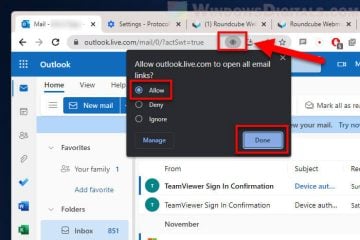The image depicts a Google Chrome browser window with multiple tabs open. The focus is on a specific tab displaying the Outlook email web interface. The upper left corner of the browser window is prominently shown, highlighting key interface elements such as the Home, View, and Help tabs, alongside a blue mail icon indicative of the email platform.

Within the Outlook web interface, a red arrow directs attention towards the URL bar, where a dropdown menu is visible. This dropdown menu prompts the user with the message: "Allow Outlook.live to open all email links", accompanied by a blue "Allow" button. Both the "Allow" button and a subsequent "Done" button are highlighted with red rectangular boxes, emphasizing the necessary steps a user should take to enable this function. 

The background is dominated by the recognizable blue and white design of Outlook, displaying sections for Home, View, Help, Favorites, Folders, and Inbox. Some example emails, including a "TeamViewer sign-in confirmation", are visible in the inbox list, adding context and realism to the instructional focus of the image. The overall aim of the image appears to be educational, guiding users on how to permit Outlook to manage email links within the browser.